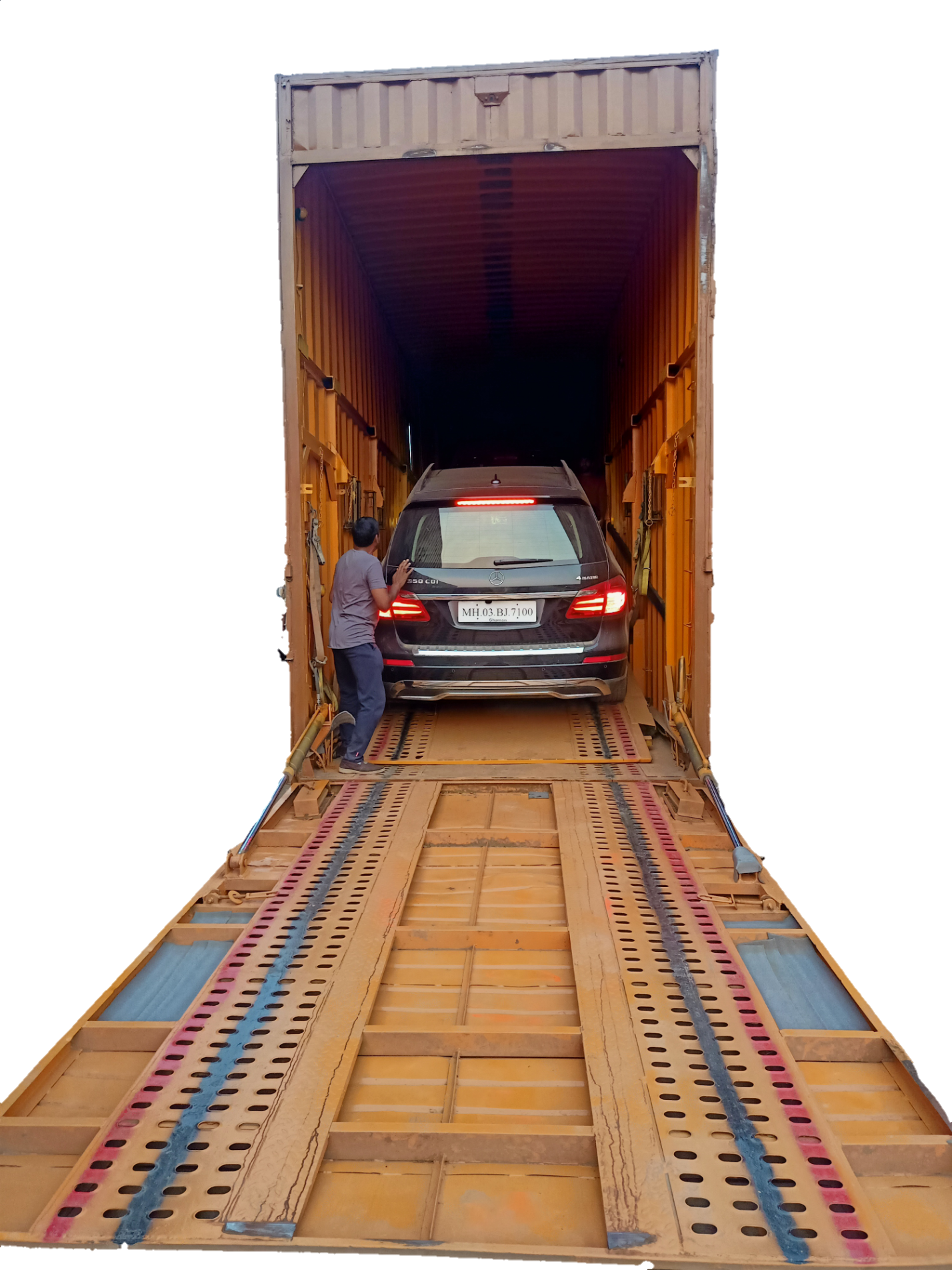The edited photograph features a black estate-style car with its brake lights illuminated, suggesting recent movement. The car is centrally positioned inside a large, old-looking container with a lowered ramp door, hinting that it was driven inside. The metal container, painted in a dull orange color with signs of wear and rust, reinforces its probable usage for long-distance vehicle transport, possibly by sea. A man, dressed in dark blue trousers and a gray top, stands directly behind the car, seemingly guiding it into the narrow, garage-like container, beyond which the interior remains too dark to discern. The scene's stark white background isolates and emphasizes the central elements, a common visual effect in product photography.